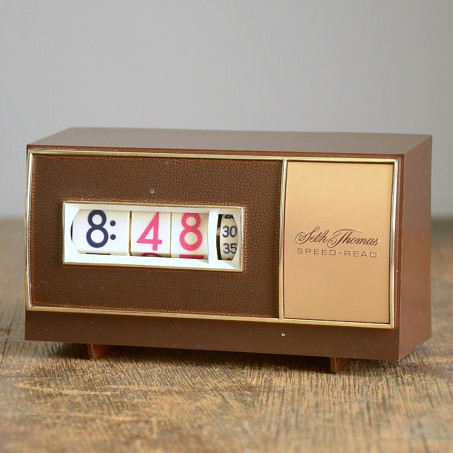The image features a retro-style, boxy alarm clock resting on a light brown wooden table. The clock is housed in a rectangular, brown plastic casing with two short, wide legs at the bottom, elevating it slightly above the table surface. The clockface exhibits an old-fashioned design, reminiscent of a vintage television set with a dark brown frame. On the left side of the clockface, there is a small window displaying the time in bold numbers: the hour digit is black, and the minute digits are pink. To the right of this, a smaller window shows the seconds in black. Towards the far right, set against a gold background, the text "Seth Thomas" is prominently displayed with "Speed Read" written below it. The overall appearance delivers nostalgic charm, blending practical timekeeping with a touch of vintage aesthetics.